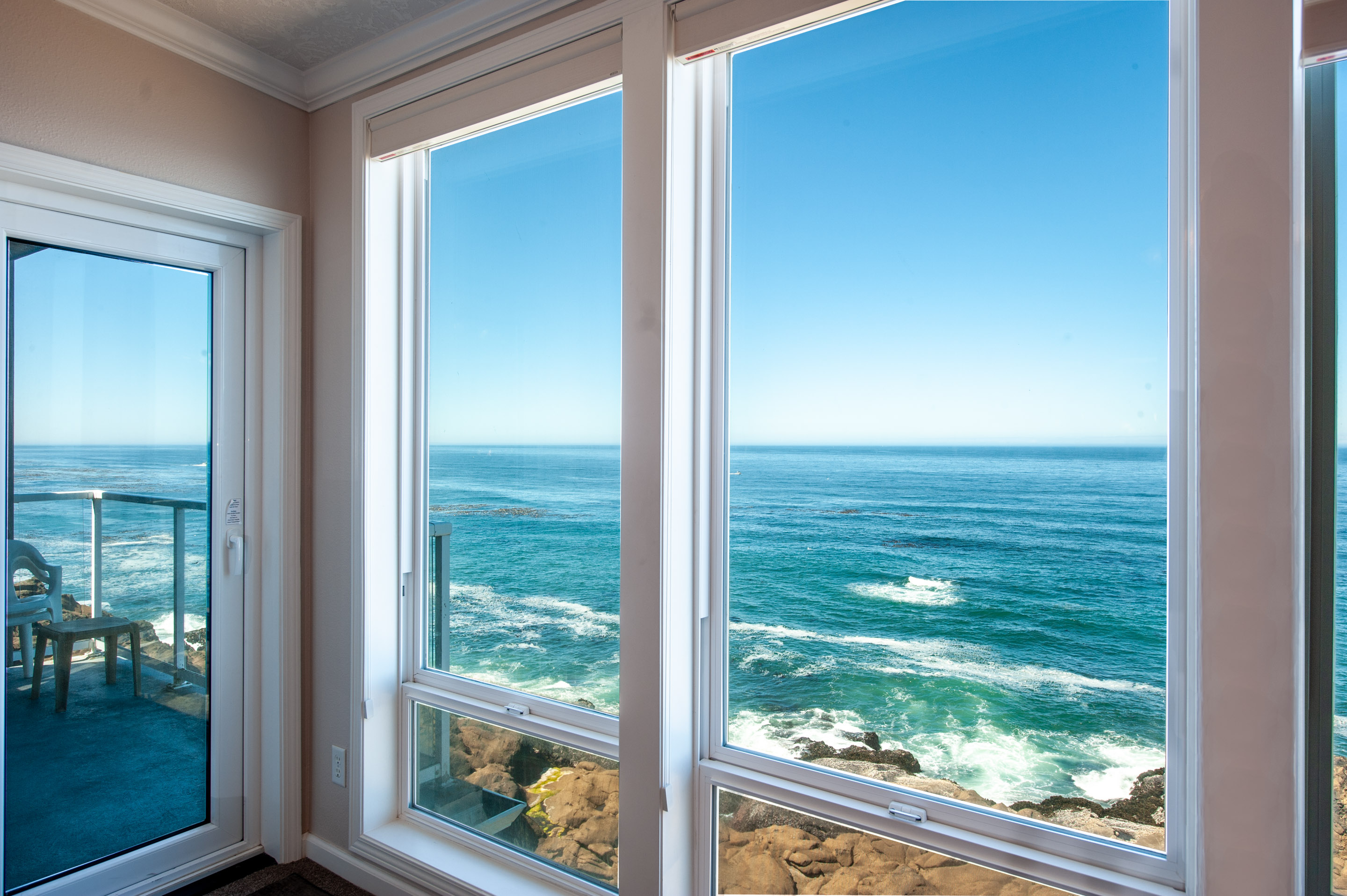The photograph captures an interior view from a beach house room, looking out towards the ocean through two large, floor-to-ceiling windows framed in peach-pink. The walls inside the room share the same pinkish hue. Directly beneath the windows lie a series of tan-brown rocks where waves crash and create white foamy pools, blending into the greenish-blue sea. The horizon is visible through the glass, showcasing a serene sky that fades from white near the horizon to light blue at the top. To the left of the windows is a glass-paneled door, also framed in white, which leads out onto a deck. The deck features a concrete floor, a sturdy silver railing, and scattered furniture, including a table and several stacked chairs. The windows have a unique design: the bottom panes are small, horizontal rectangles, while the top panes are large and vertical, enhancing the view of the tranquil ocean setting.